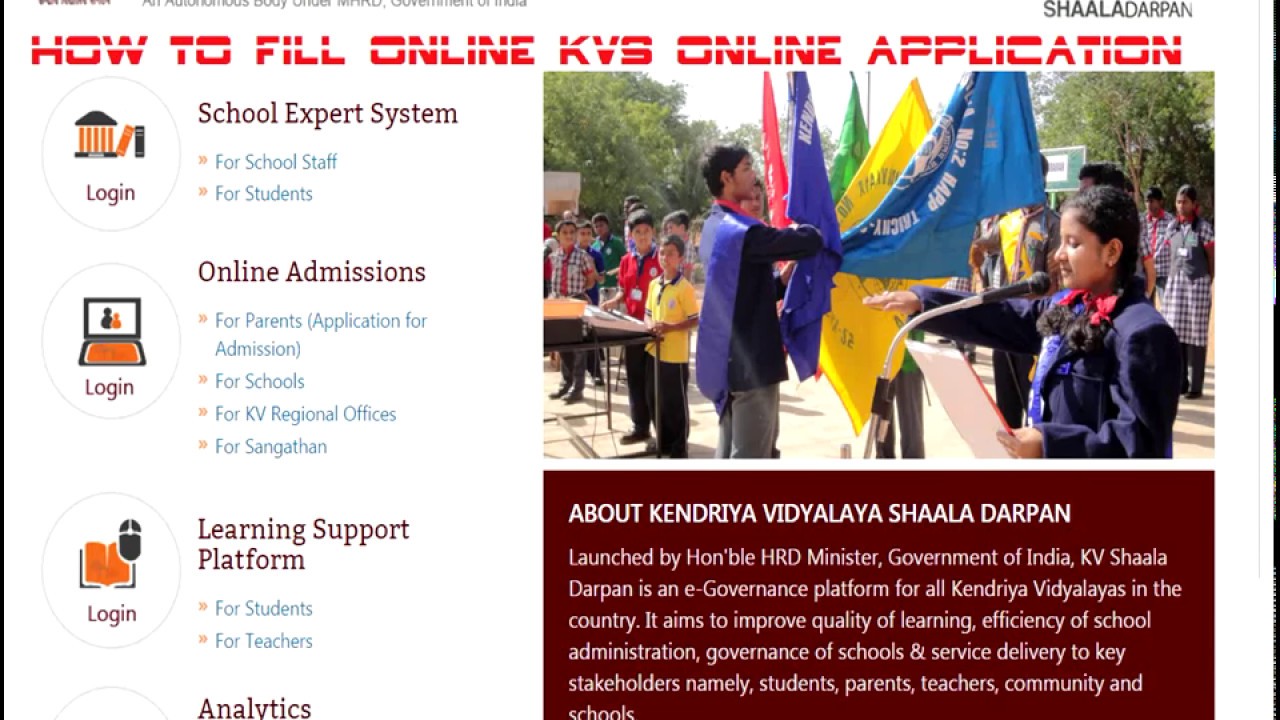In the image, there's a prominent title "SHAALA DARPIN" in bold, set against a white background. The top section features the text "How to Fill Online KVS (Kendriya Vidyalaya Sangathan) Application" with "KVS" in all capitals. Below this, the phrase “School Expert System” appears in purple, followed by "For School Staff" in blue. 

For students, the term "Online Admissions" is highlighted in purple, and "For Parents" is in blue, with the additional note "(Application for Admissions)" beside it. The section indicates that the admissions are pertinent to KVS regional offices and schools.

Additional informational text mentions "KVS (Kendriya Vidyalaya Sangathan) Learning Support Platform" in purple, aimed at students and teachers, with “Analytics” in purple. 

To the right side of the image, there is a photograph of young students, possibly college-aged or younger, with a young girl appearing to give a speech. Several flags can be seen in the background. A red rectangle contains white text that states "About Kendriya Vidyalaya Sangathan SHAALA DARPIN."